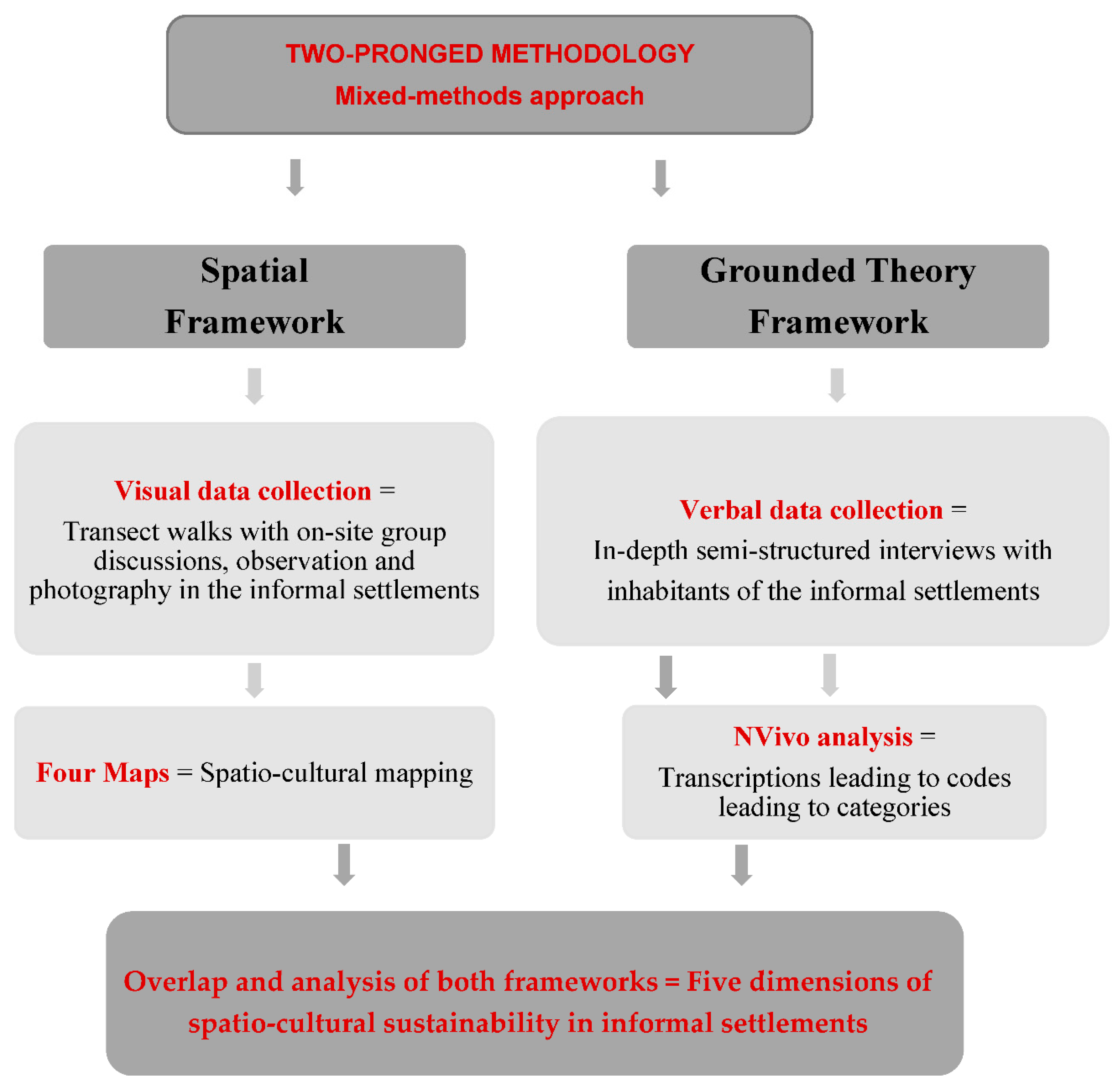The image is a detailed flowchart with a white background and features rounded gray boxes connected by arrows, forming a structured hierarchy. At the top center, a large gray rounded box with red text reads, "Two-Prong Methodology, Mixed Methods Approach." This box branches into two sides, each detailing different frameworks.

On the left side, a sequence of gray rounded boxes describes the "Spatial Framework." The first box underneath it reads "Visual Data Collection," followed by "Transect Walks with On-Site Group Discussions." An arrow leads to the next box that says "Four Maps Equal Spatial Cultural Mapping."

On the right side, a similar sequence unfolds under the "Grounded Theory Framework." The initial box states "Verbal Data Collection," succeeded by another emphasizing the processes: "NVivo Analysis, Transcriptions Leading to Codes Leading to Categories" in red text.

Both sides converge at the bottom into a larger, more expansive gray rounded box, marked in bold red text: "Overlap and Analysis of Both Frameworks Equal Five Dimensions of Spatiocultural Sustainability in Informal Settlements." The flowchart is purely textual with no other images, symbols, or colors apart from the mentioned gray boxes and red text.